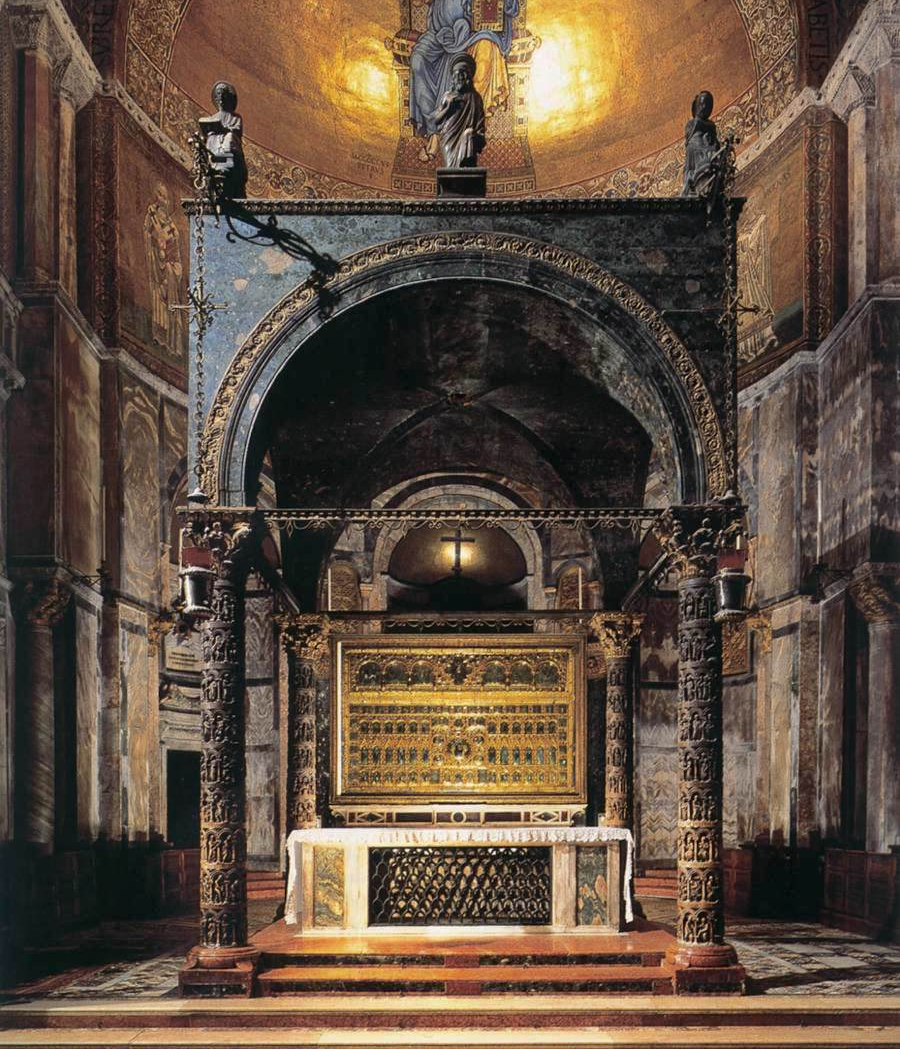The photograph captures the interior of a grand, ancient, gothic-style cathedral with large stone walls adorned with intricate religious carvings. Central to this cathedral is an elaborate altar situated beneath a magnificent gold-tinted domed ceiling. The altar stands on a base supported by four dark gray pillars, each intricately carved with detailed designs. Above these pillars is a vast archway with a flat top, outlined with a gold inlay trim, and adorned with sculptures of religious figures, including a statue of Jesus at its apex.

In the center beneath this grand architectural structure, a large table covered with a pristine white cloth holds a prominent, shiny golden box. This box, with its square paneling, gleams brightly, drawing attention amidst the intricately carved surroundings. The cathedral's flooring appears to be made of stone or marble, complementing the overall solemn and historic ambiance of the sacred space.